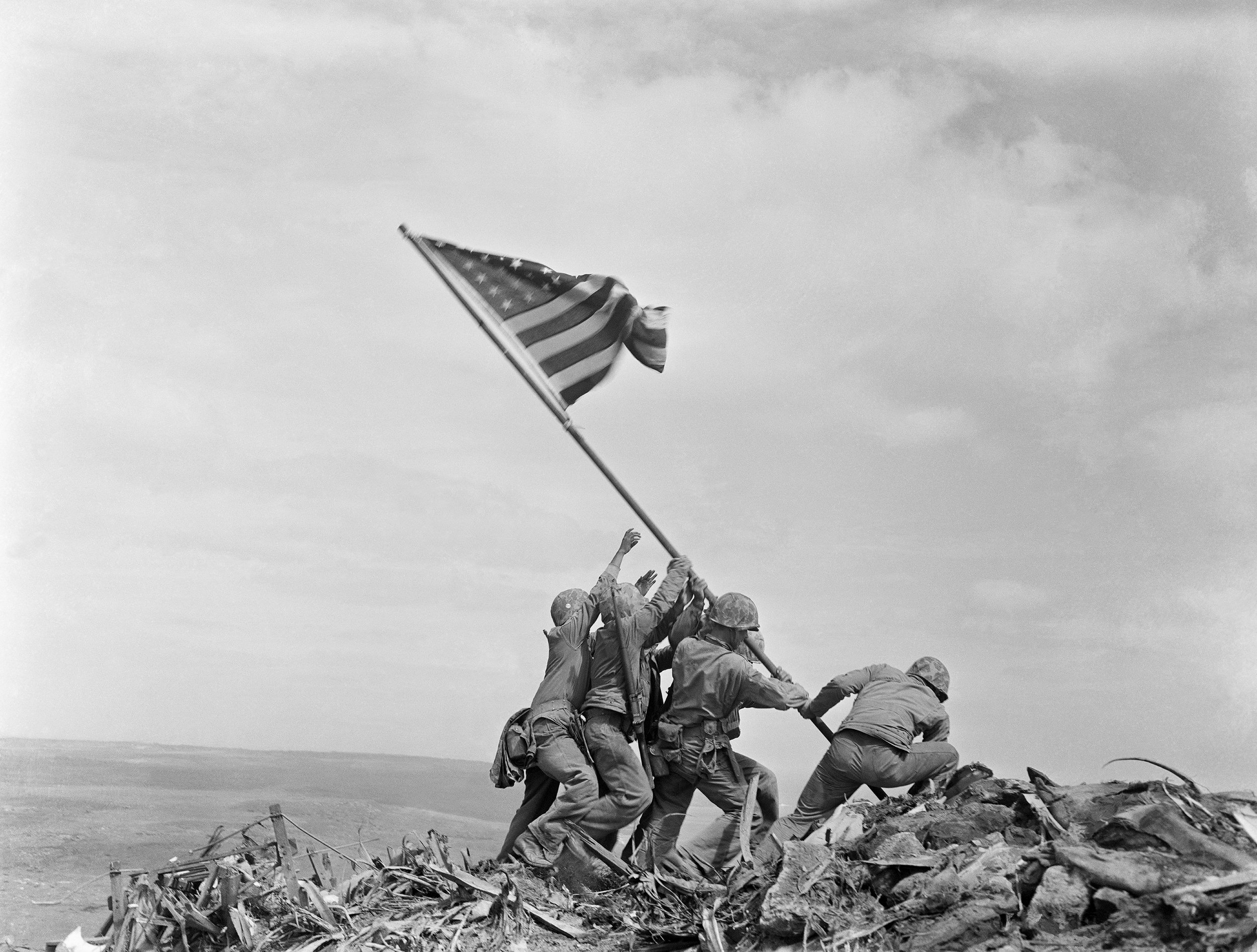This is a black and white photograph, reminiscent of an old-time image, capturing a historic scene where five soldiers, possibly from the army, are shown in an effort to plant the American flag. The scene is set against a backdrop of a cloudy sky, with thick white clouds vividly discernible. The ground beneath the soldiers is a rough terrain strewn with rocks, sticks, and debris, resembling the ruins of machinery. In the distant background, a calm, flat body of water, likely an ocean, stretches out towards the horizon. The soldiers, clad in camouflage helmets akin to those from World War II, are intently focused on securing the flagpole into the challenging ground. The flag itself, adorned with stars and stripes, is depicted waving in the breeze, poised to stand tall once firmly planted. The composition and the determined posture of the soldiers evoke a sense of historical importance and patriotic determination.